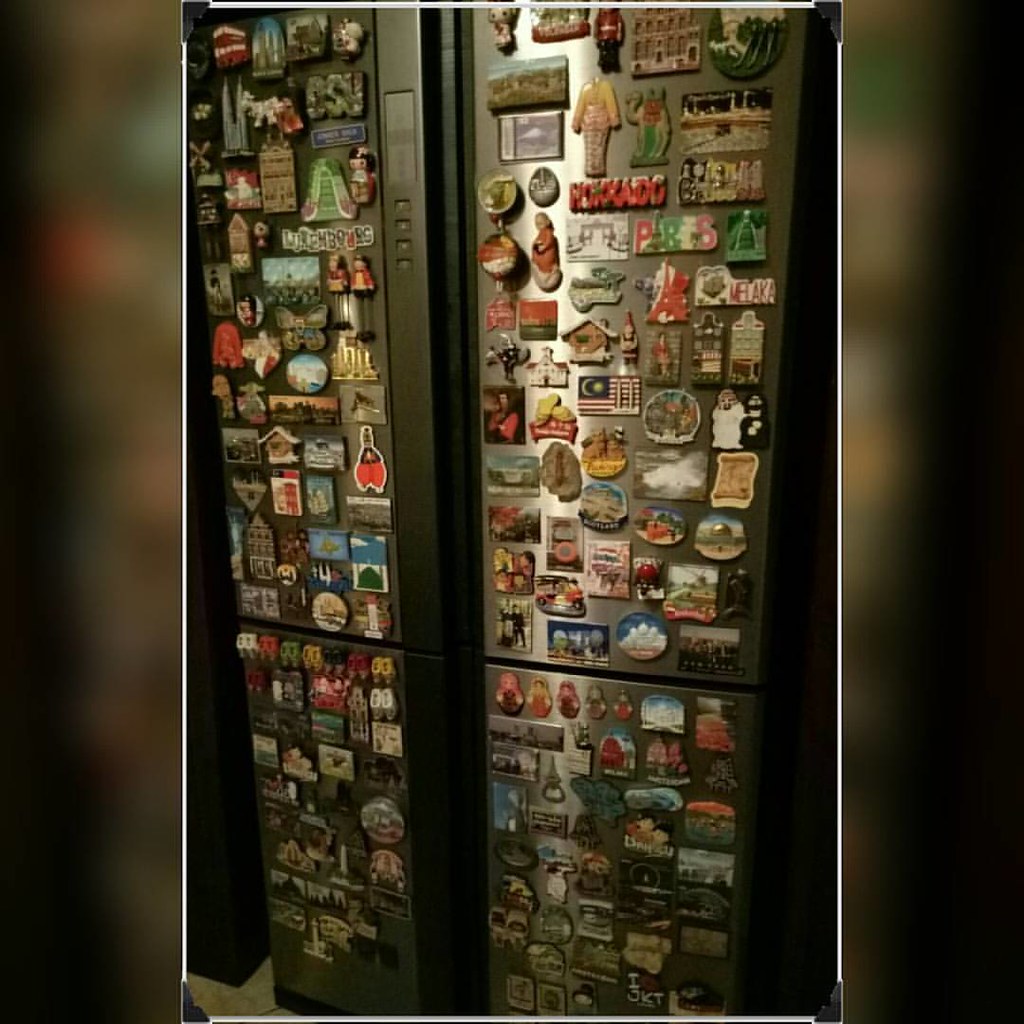The image depicts a high-end, stainless steel, four-door refrigerator and freezer combination. The fridge is entirely covered with an extensive collection of around 200 refrigerator magnets of various shapes, sizes, and colors, ranging from square and round to more intricate designs. Many magnets feature names and images of international locations, such as Paris, Malacca, and Luxembourg, suggesting they are souvenirs from the owner’s travels or aspirations. Among them, specific items like a motor scooter, a set of Russian nesting dolls, OSU (likely Ohio State University) memorabilia, and a variety of flags highlight the diverse nature of the collection. The magnets are thoroughly scattered across the fridge, leaving hardly any unoccupied surface. The photograph is taken slightly from the right, capturing the center part of the refrigerator in focus while the sides are blurred, emphasizing the colorful and detailed presentation of the magnets against the metallic backdrop.